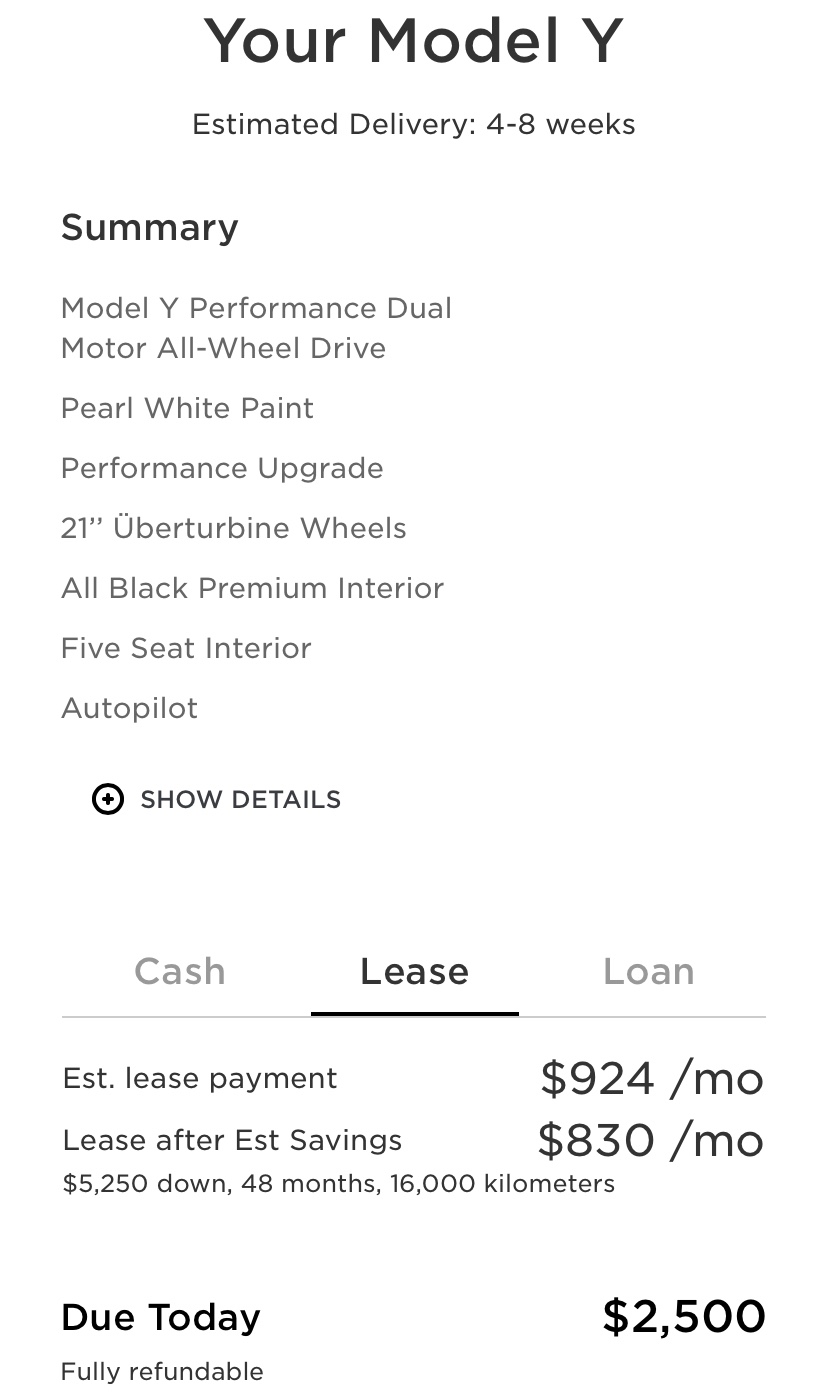A screenshot capture of an order form for a Tesla Model Y displayed in portrait orientation on a white background, without defined edges. 

At the center of the image, bold black text states, "Your Model Y," with the subtext, “Estimated delivery: 4-8 weeks,” in a smaller font beneath. 

Below, a "Summary" section in gray lists key specifications: 

- Model Y Performance
- Dual Motor All-Wheel Drive
- Pearl White Paint
- Performance Upgrade
- 21-inch Überturbine Wheels
- All Black Premium Interior
- Five-Seat Interior
- Autopilot

A plus sign followed by "Show Details" is located under the specifications. Next, a light gray box containing text and additional options is visible, with a thin gray line running horizontally across to separate clickable categories: "Cash" (grayed out), "Lease" (highlighted in black and underlined), and "Loan".

The "Lease" option is selected, showing the following details in black text: 

- Estimated lease payment: $924 per month
- Lease after estimated savings: $830 per month
- Down payment: $5,250
- Lease term: 48 months
- Kilometer allowance: 1,600 km per month

Further down, in black text, "Due today: $2,500" is noted, with "Fully refundable" written in gray underneath, indicating someone is reviewing the lease terms for a potential car lease.